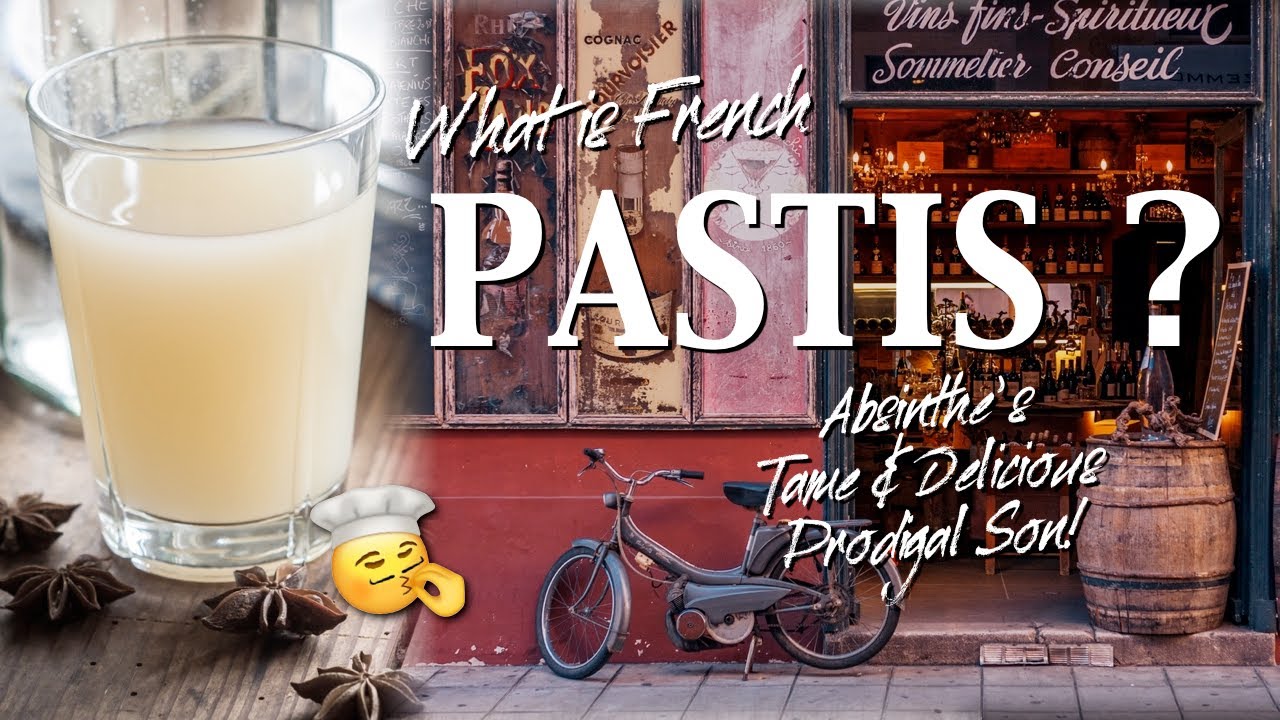The image showcases a charming and picturesque French storefront, indicating it is a wine or liquor store with a sign that reads "Vins Fins Spiritueux Sommelier Conseil." Superimposed on the image is large white text in two different fonts, asking "What is French pastis, absinthe's tame and delicious prodigal son?" To the left of this text is a glass containing a milky white liquid, placed on a wooden table with star anise arranged around it, suggesting the drink's anise flavor. Adjacent to this setup is a chef's kiss emoji, enhancing the appeal of the drink. In front of the red-colored store, there is an old-fashioned bicycle leaned against the front, and a barrel holding a sign at the entrance, adding to the quaint and inviting atmosphere.